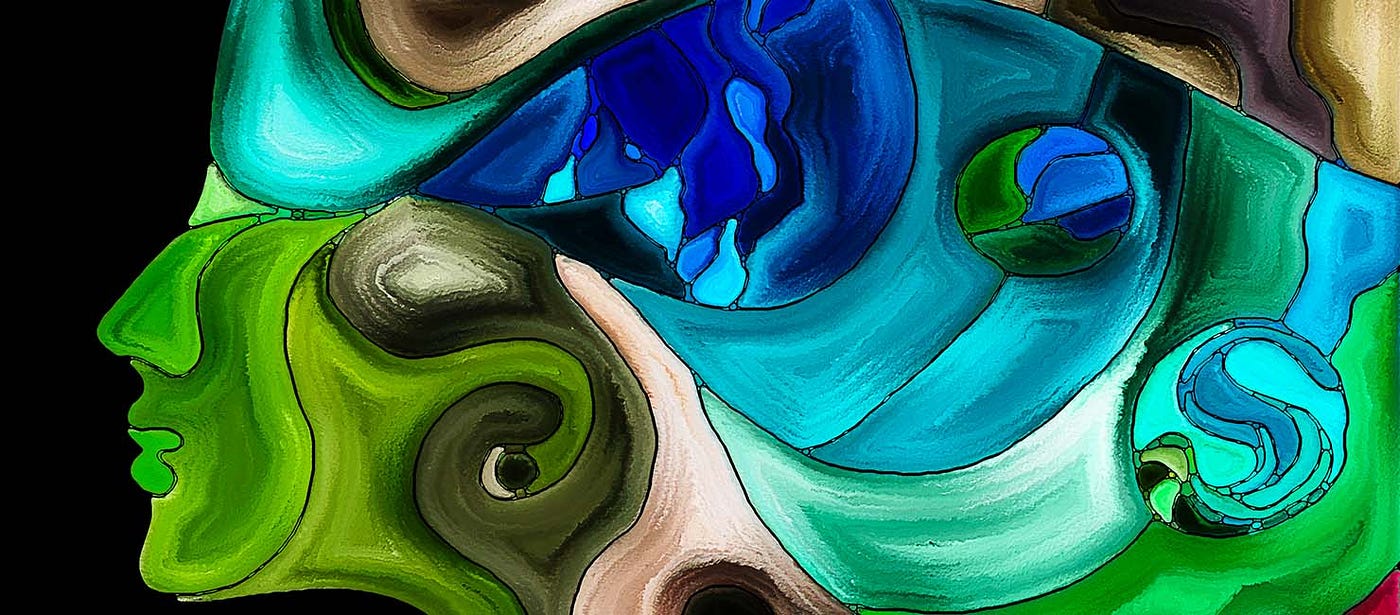In this vibrant and striking abstract piece of art, the image bursts into a spectrum of greens and blues, ranging from deep green, chartreuse, and light green to soft sky blue and brilliant sapphire blue. This colorful cacophony defines the contours of a stylized face on the left side: the green hues collectively shape a nose, lips, and jawline, while the varying blue tones above suggest a mass of hair sweeping across the forehead and flowing to the right. Against a backdrop of negative space in black on the left, the intricate pattern transforms into an array of swirls and interlocking shapes. Adding to this complex palette, there is a scattering of whites, grays, browns, and tans, forming layers that echo the facial structure. Multiple circles and more undefined shapes weave deeper into the piece, underscoring the abstract nature of the composition. The entire artwork, with its intertwining designs and dynamic color scheme, invites the viewer into a mesmerizing interplay of form and color.